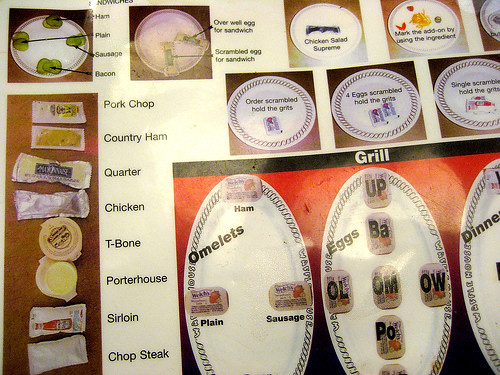This instructional board appears to be a teaching tool used in a restaurant setting, likely to guide kitchen staff on meal preparation and plating. On the left side of the board, there is an illustrated plate with pickles arranged in a clock-like formation, each adorned with arrows and labels: "ham" at the top, "sausage" at three o'clock, "bacon" at six o'clock, and "plain" at nine o'clock. This seems to indicate different ways to serve pickles with specific meats. Below this pickle plate, a row of condiment containers is displayed, featuring mustard, mayo, butter, and ketchup, presumably to instruct staff on appropriate condiment pairings.

Adjacent to this setup, a detailed list enumerates various entrees: pork chop, country ham, quarter chicken, T-bone, and porterhouse sirloin. Additionally, there is another plate illustration dedicated to omelets, organized similarly to the pickle plate, with labels for "ham," "plain," and "sausage." Further notations on the board include "eggs up," "bacon omelet," "eggs scrambled," "hold the grits," and "chicken salad supreme," providing clear guidance on meal compositions and sequencing. This visually structured board serves as a comprehensive reference for the precise assembly and presentation of dishes.